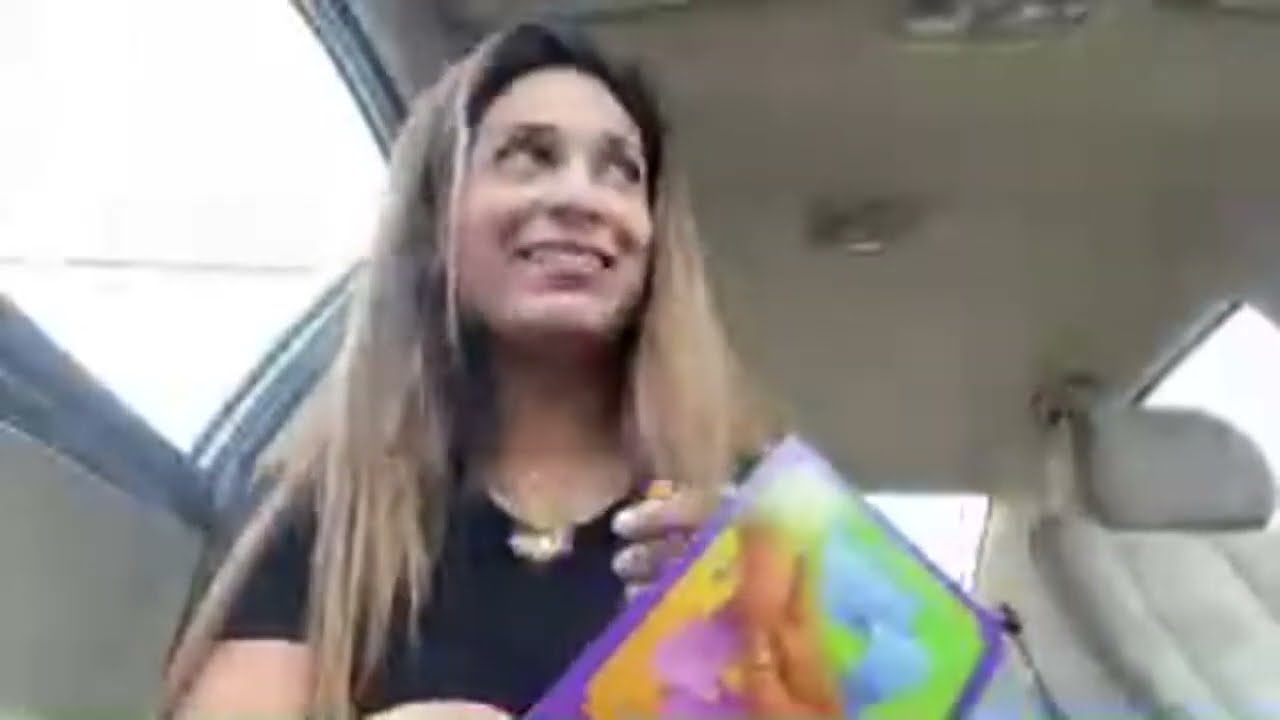The image depicts a blurry, out-of-focus view of a young woman sitting in the front passenger seat of a vehicle. The shot is angled upwards, likely from her lower leg area, capturing her face tilted slightly to the left with a half-smile. She has long, light brown to blonde hair with some darker roots and streaks, and she is wearing a short-sleeved black shirt. The interior of the car features a white or light gray upholstery and ceiling, with a visible dome light. Sunlight streams through the windows, creating a bright background that suggests it's daytime. The woman holds a colorful item in her hand, featuring hues of blue, yellow, green, purple, and possibly orange, though its exact nature is unclear. The overall composition includes a mix of tan, black, green, and other vivid colors, enhancing the scene despite the photo's lack of clarity.